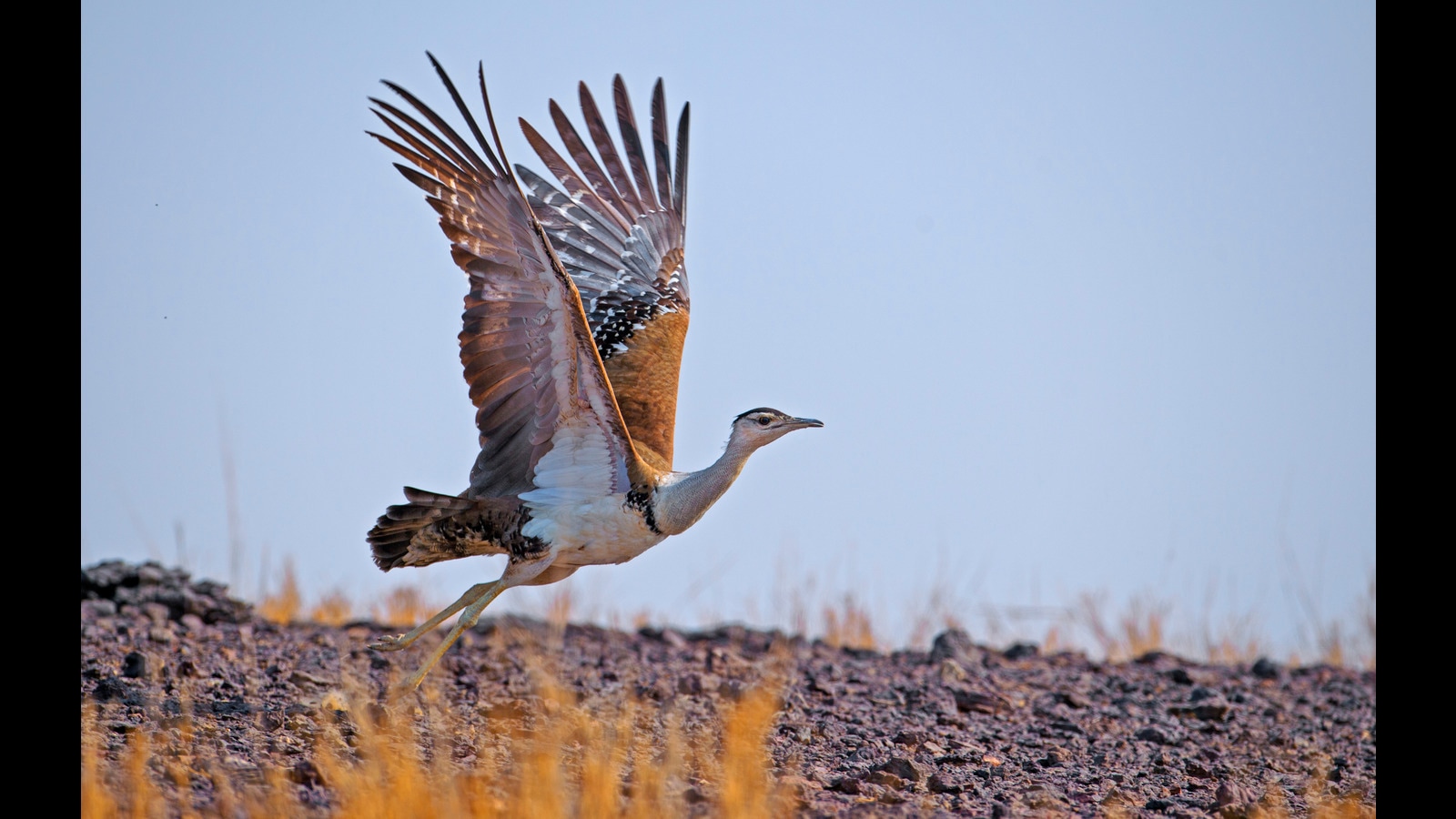In this crisp and vibrant photograph, a grand bird with a commanding presence is captured just moments before taking flight in a stark, desert environment. The bird, with its extensive wingspan and elongated beak, is perched on a rocky, gravel-strewn hill accented by golden, dead grasses and brush. Its feathers showcase a striking palette of burnt orange, gray, and light white on the underbody, complemented by various shades of brown. The image details the bird's poised posture, with wings upright and ready for a downstroke, as it gazes to the right. The clear, unclouded blue sky forms a serene backdrop, enhancing the focus on the bird. Encased by black banners on the left and right, the photograph offers an undisturbed view of this majestic creature, capturing the barren, sunlit landscape in the background.